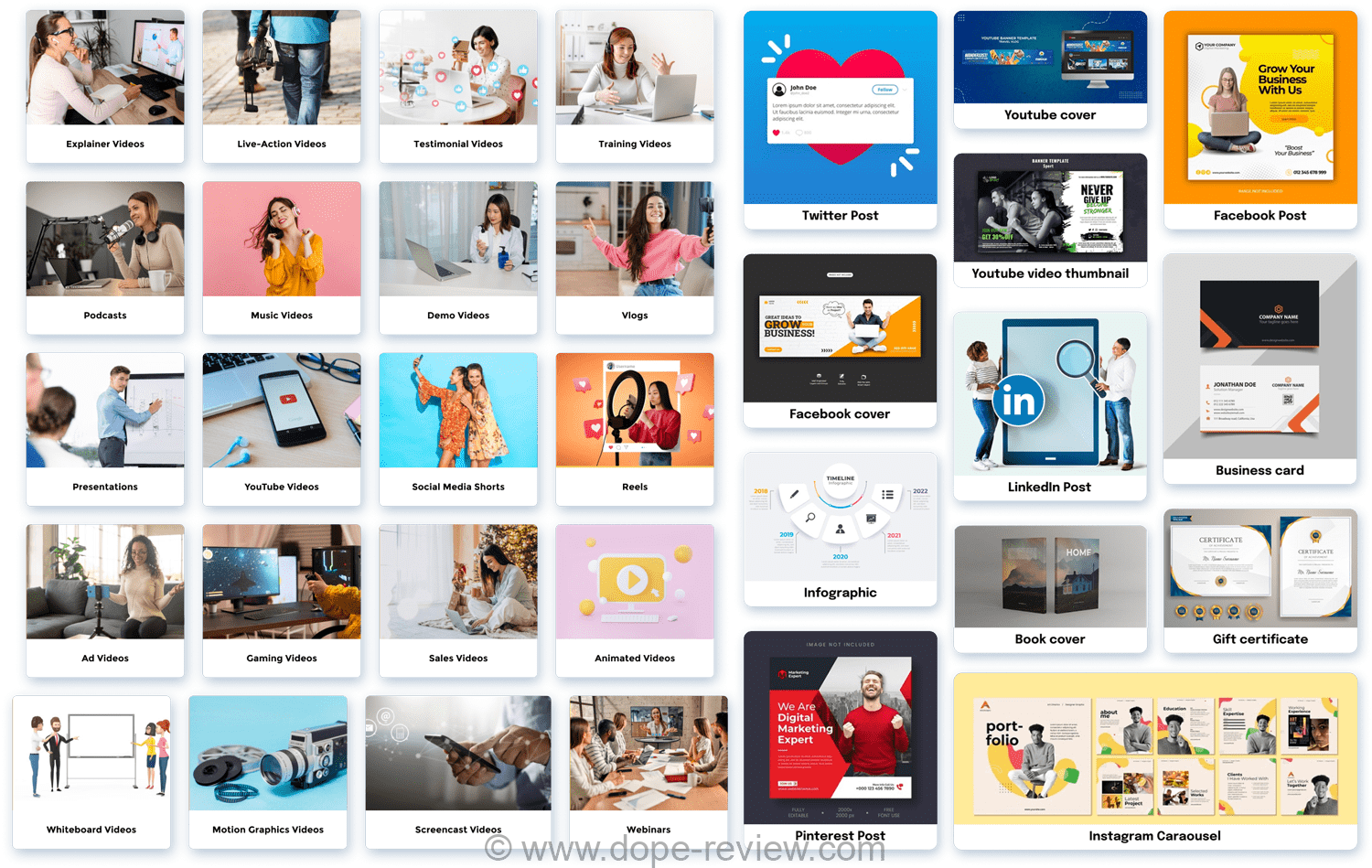This screenshot captures a webpage displaying various visual content categories arranged in a systematic layout. The left side showcases a detailed 4x5 grid containing twenty different types of video content, each represented by a thumbnail followed by a white-bordered label. These categories include explainer videos, live action videos, testimonial videos, training videos, podcasts, music videos, demo videos, vlogs, presentations, YouTube videos, social media shorts, reels, ad videos, gaming videos, sales videos, animated videos, whiteboard videos, motion graphics videos, screencast videos, and webinars. On the right side, a more conventional grid structure features additional media types: Twitter posts, YouTube cover, Facebook posts, YouTube video thumbnail, and Facebook cover. The design effectively categorizes a broad range of content types, making it easy for users to locate and identify the specific format they need.